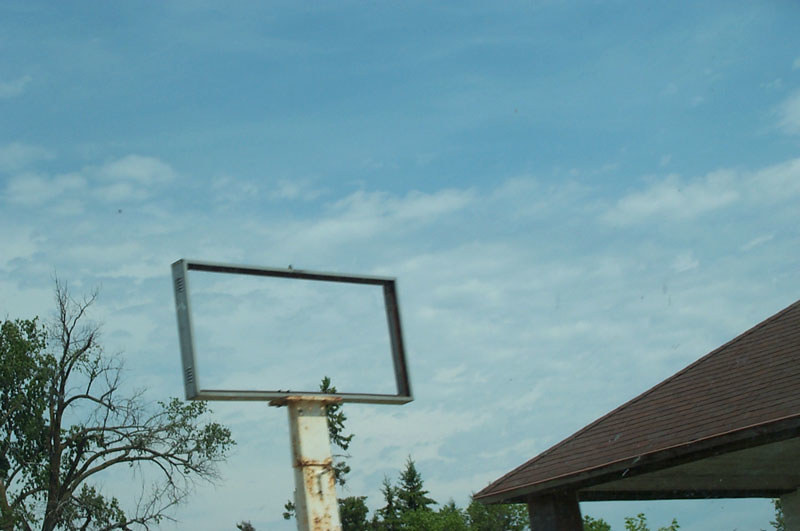In this slightly blurry daytime photograph, the vast majority of the frame is dominated by a serene blue sky interspersed with patches of white cloud cover. In the lower right corner, the top of a tree peeks into view, while the lower left corner reveals a portion of the roof of an open-air gazebo. The main focus of the image is an empty billboard frame, mounted on a large, rusty white pole. Notably, the rectangular metal structure is devoid of any signage, allowing the blue sky to be seen right through it. Adding a touch of life to the scene, a small bird is perched atop the vacant billboard frame, seemingly surveying its airy domain.